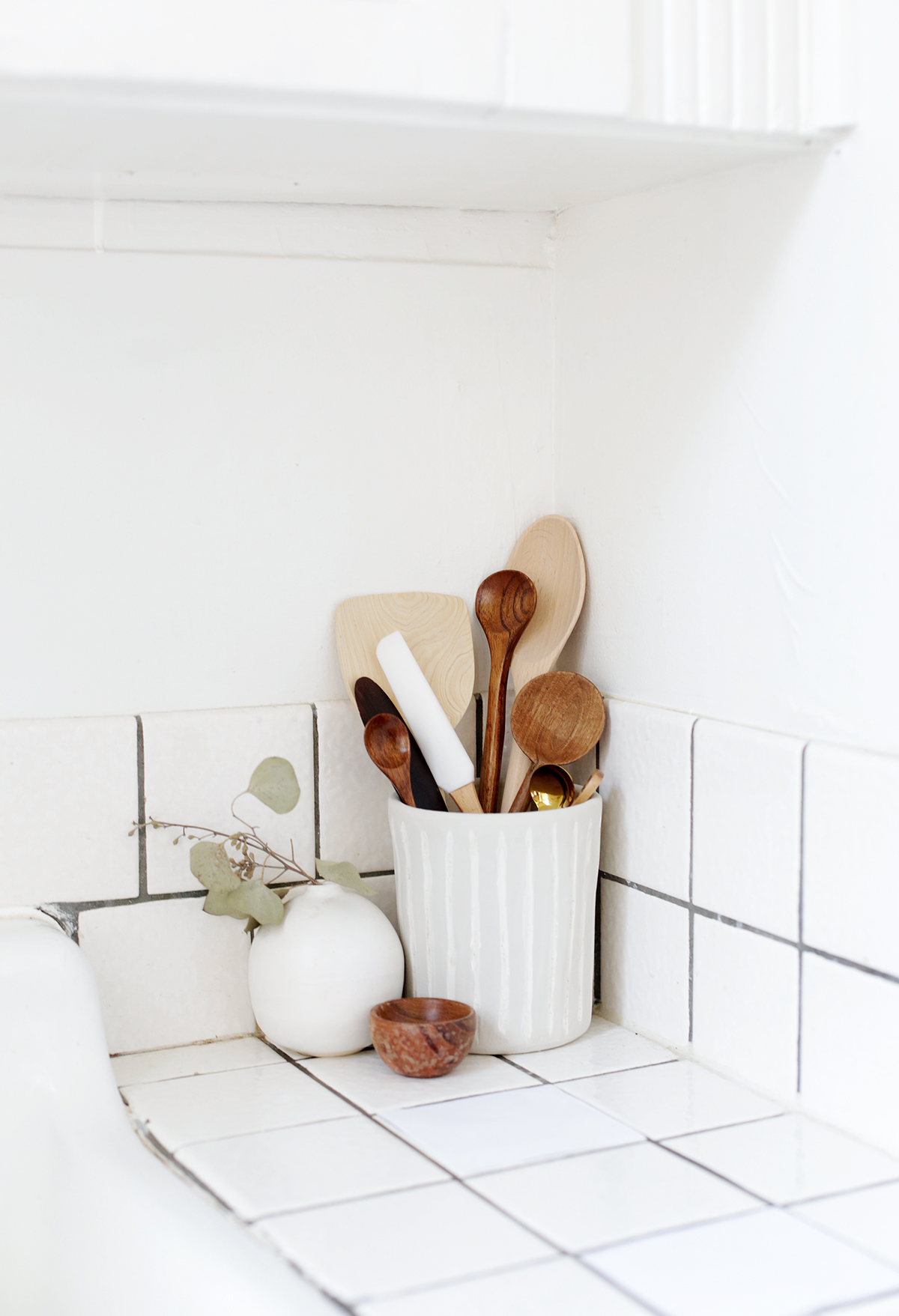This image captures a pristine, minimalist corner of a white kitchen, featuring a classic yet simplistic design with its white tile countertop and matching white tile backsplash, accented by gray grout. The tiles, which are square rather than subway style, extend up the wall two tiles high, meeting a plain white painted wall above it. In the spotlight of this cozy kitchen corner is a white, lidless canister filled with a variety of wooden utensils, including spoons, spatulas, and a golden measuring spoon. The utensils come in different shades, from dark brown to light tan. Next to the utensil holder sits a small, spherical white vase holding a dried eucalyptus plant, adding a touch of natural elegance. In front of the vase is a tiny brown wooden bowl, completing the scene on this neat and clean tiled counter. The whole setup is situated adjacent to what appears to be a white ceramic sink, highlighting the kitchen's clean and classic aesthetic.